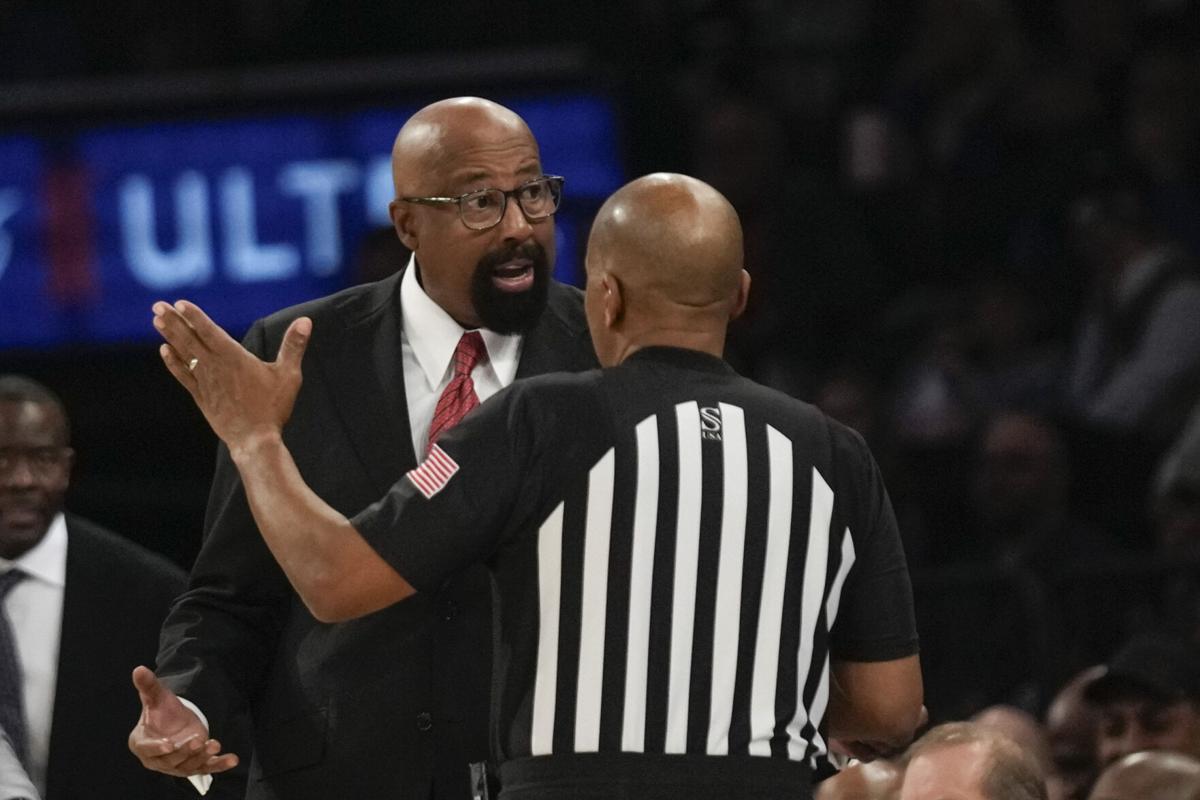In this image, a heated moment during a sporting event is captured with two main figures prominently featured in the center. Both individuals are African American men seemingly engaged in an argument. The man on the left, likely the referee, has his back to the camera, but his raised left hand and expressive body language suggest he is making a point. He is dressed in a black shirt with white stripes, reminiscent of a referee's uniform, and has a red and white flag on his left arm, indicating his official role. The other individual appears to be a coach, discernible by his attire—a black suit, white shirt, and a distinct red necktie. He faces the camera with a stern expression, clearly involved in the dispute. In the background, we can see spectators observing the scene and a blue-highlighted sign with the letters "ULT," adding context to the event's branding or sponsoring entity. The atmosphere is charged, reflecting the intensity typical of competitive sports environments.